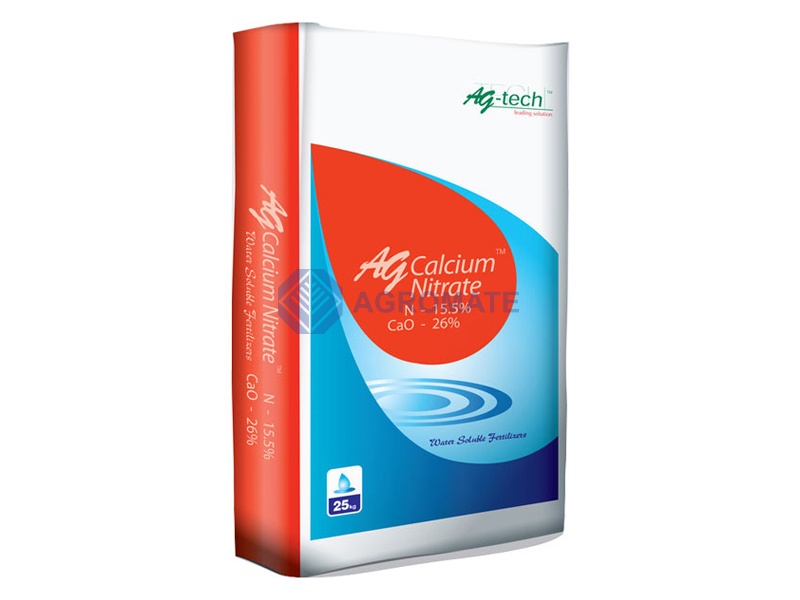The promotional image features a white box of calcium nitrate prominently branded as "AG Calcium Nitrate." The front of the box displays a detailed design: a bright orange teardrop icon centrally placed on a blue background, within which the title "AG Calcium Nitrate" is boldly written in white. Underneath, smaller text reads "Water Soluble Fertilizers" in cursive blue letters. In the top right corner, the company logo, "AG-Tech," appears in green text accompanied by a horizontal green line and small red text beneath it. A graphic depicts a red droplet falling into blue water, creating a ripple effect, with "AG Calcium Nitrate N-15.5% CaO-26%" inscribed inside the red droplet.

The bottom left corner of the front side features a white square showcasing a water droplet icon and a blue box containing the weight "25 kg." The left side of the box is entirely red with white text stating "AG Calcium Nitrate" at the top, followed by "N-15.5%" in larger font. Additional smaller, less legible text follows on the second row. A watermark with the letters "A-G-R-O-M-A-T-E" is superimposed on the entire image for branding.